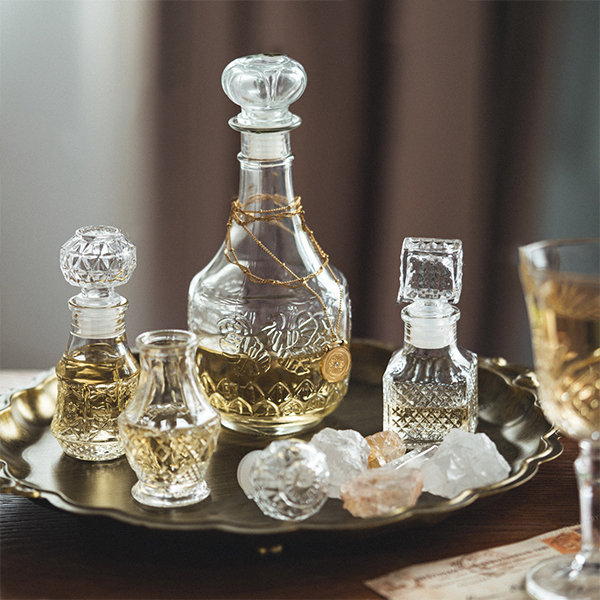This detailed color photograph captures an elegant tabletop scene, featuring a scalloped black tray placed centrally. On the tray, there are four distinct, antique-style crystal bottles, each showcasing unique designs and elaborate stoppers. The largest decanter, stationed in the middle, is etched with an intricate, possibly floral, pattern and tied with a rusted gold chain around its neck. It contains a yellowish liquid, about a quarter full, suggesting it may have been used to serve wine.

To the left of this main decanter, a smaller bottle filled with the same yellowish liquid sits neatly, while another similar bottle nearby has its stopper removed and placed on the tray. To the right, there is a petite decanter with a square top. Each of these bottles exemplifies fine craftsmanship, with designs that evoke a sense of antiquity and elegance.

An assortment of crystal objects adorns the tray, adding to the luxurious display. In the foreground, slightly out of focus and resting on what appears to be an old piece of mail, is a wine glass filled with white wine. This glass, half cut-off by the photograph's edge, subtly complements the tray's sophisticated assembly, evoking a timeless and refined atmosphere.